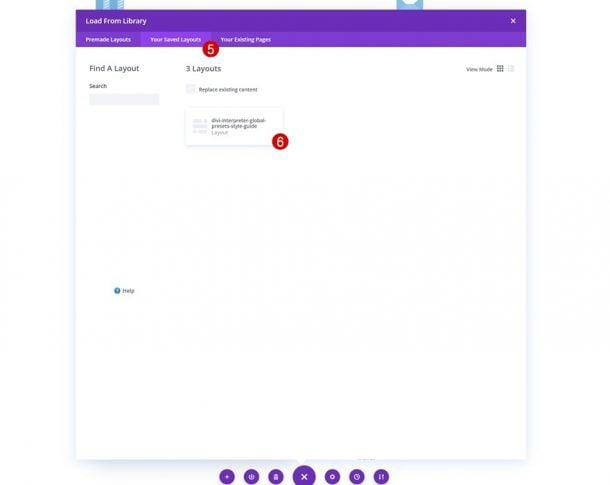**Caption:**

The image displays a user interface with a low resolution. In the upper-left corner, there is a purple strip with the text "loaded from library" while the right side features an 'X' icon. Below this are three tabs highlighted in purple with white text, although the specific details are blurry. Between the tabs labeled as something layouts and your something pages, there is a red circle with a white number '5' inside it.

The background is predominantly white. On the left side, the UI includes a "find a layout" label followed by a gray, empty search data field. Adjacent to this, on the right, it reads "three layouts" next to a gray box with text that appears to say "replace," though the accompanying words are unreadable. There is another box nearby with indistinguishable writing. In the bottom right corner of this section, a red circle contains a white number '6'.

To the far right, the interface has a "view mode" button represented by nine small squares forming a larger square. At the bottom left corner, there seems to be a "help" option. Below the central field, a purple circular button with an 'X' is located in the middle, flanked by three additional buttons on either side.